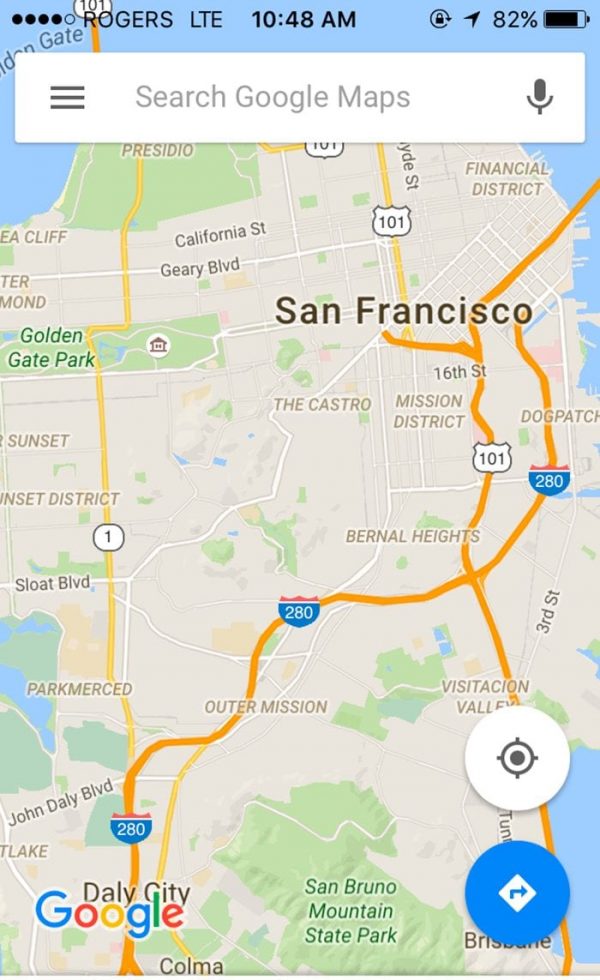This is a detailed screenshot of a Google Maps view captured on a cell phone. The status bar at the top left indicates that the user has four bars of cellular coverage with Rogers LTE, the time displayed is 10:48 AM, and the battery life stands at 82%. A white search bar is prominent at the top of the screen, with three horizontal black lines on the left, indicating the menu. The text "Search Google Maps" is centered within the search bar, and a microphone icon is on the right for voice search functionality.

The map displayed is of San Francisco, with the city's name clearly visible on the right side. Notable areas identified on the map include the Financial District, The Castro, Mission District, Dogpatch, Bernal Heights, San Bruno Mountain State Park, John Daly Boulevard, Sloat Boulevard, Sunset District, Golden Gate Park, the Presidio, California Street, Geary Boulevard, Daly City, and Colma. The Interstate 280 is marked with an orange curving line across the map. At the bottom left corner, the Google logo is visible. The screenshot does not contain any human figures.